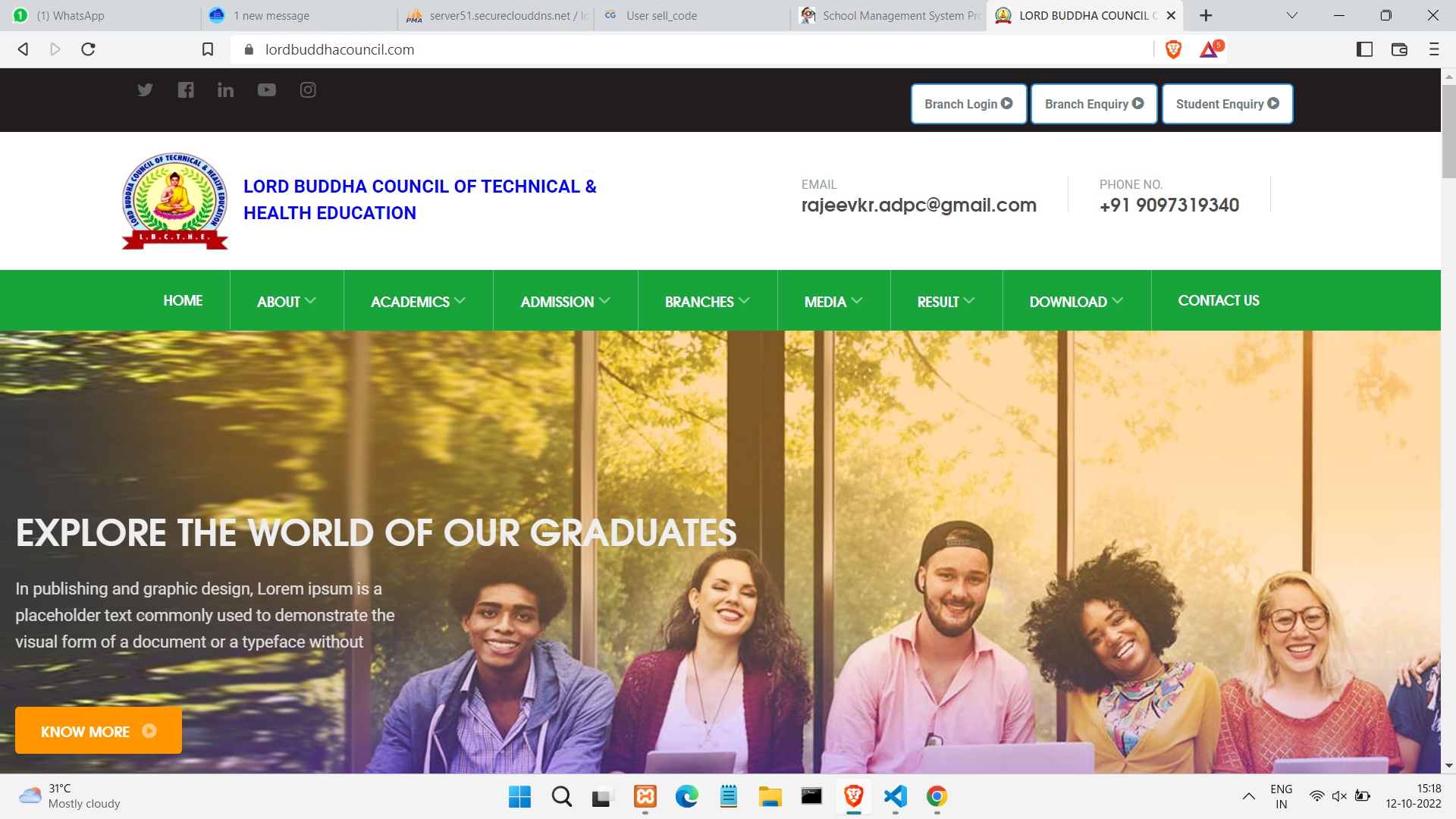The image depicts the homepage of a website with the URL displayed in the search bar as "lordbudhascouncil.com." This full name, "Lord Buddha Council of Technical and Health Education," is represented by a logo featuring a yoga Buddha figure against a yellow background, surrounded by green leaves, with a blue border and a red banner. 

At the top, a lime-green navigation bar includes tabs such as Home, About, Academics, Admission, Branches, Media, Results, Download, and Contact Us. Below this bar, the main header reads "Explore the world of our graduates," accompanied by a group photo featuring four graduates: a white woman, a black woman, a white man, and a black man.

Underneath the header, there's placeholder text explaining "Lorem Ipsum is a placeholder text commonly used to demonstrate the visual form of a document or a typeface without..." which is cut off abruptly. 

The bottom of the image displays an orange box, though its function or content is not specified.